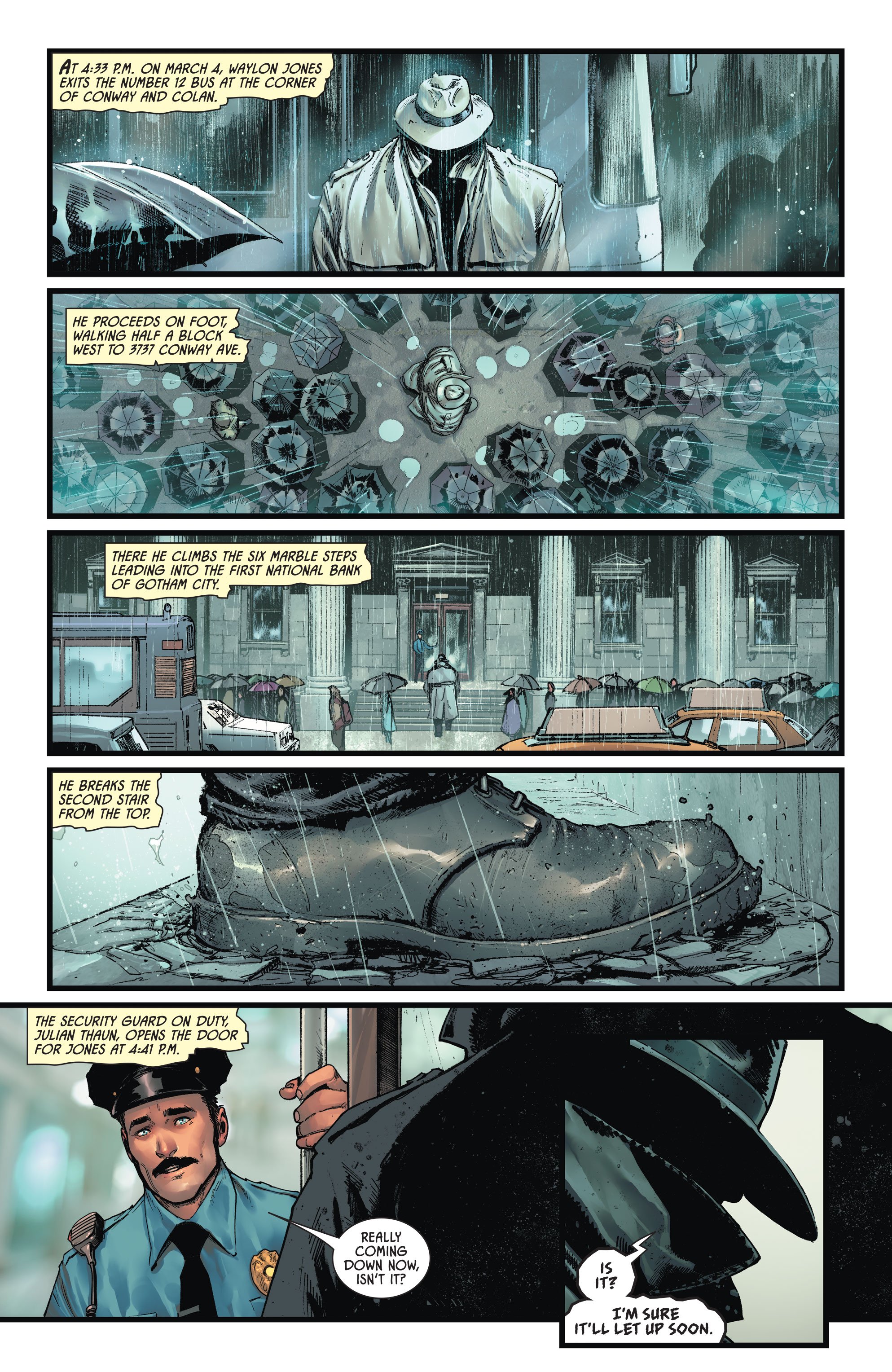A series of detailed comic book drawings depicting Waylon Jones' movements begins at 4:33 p.m. on March 4th. In the initial panel, the narration indicates that Jones exits the number 12 bus at the corner of Conway and Colan. The illustration captures a man in a raincoat and hat with an empty appearance, suggesting possible invisibility, while a bus can be seen in the background.

In the next panel, the text mentions that Jones proceeds on foot, heading half a block west to 3737 Conway Avenue. The artwork portrays him walking in the rain, hat firmly in place, surrounded by numerous pedestrians carrying umbrellas.

The following panel showcases Jones climbing the six marble steps leading into the imposing First National Bank of Gotham City. The steps glisten with rain, and passersby with umbrellas populate the scene, contributing to the city's bustling atmosphere.

A close-up in the subsequent panel highlights a significant moment: Jones' shoe stopping on the second step from the top, which he cracks underfoot.

In the final panel, the comic depicts Security Guard Julian Thaun opening the bank door for Jones at precisely 4:41 p.m. Thaun, commenting on the heavy rain, says, "Really coming down now, isn't it?" Jones replies nonchalantly, "Is it? I'm sure it will let up soon." The illustration emphasizes the rainy setting and the interaction between Jones and the guard, adding to the narrative's immersive detail.